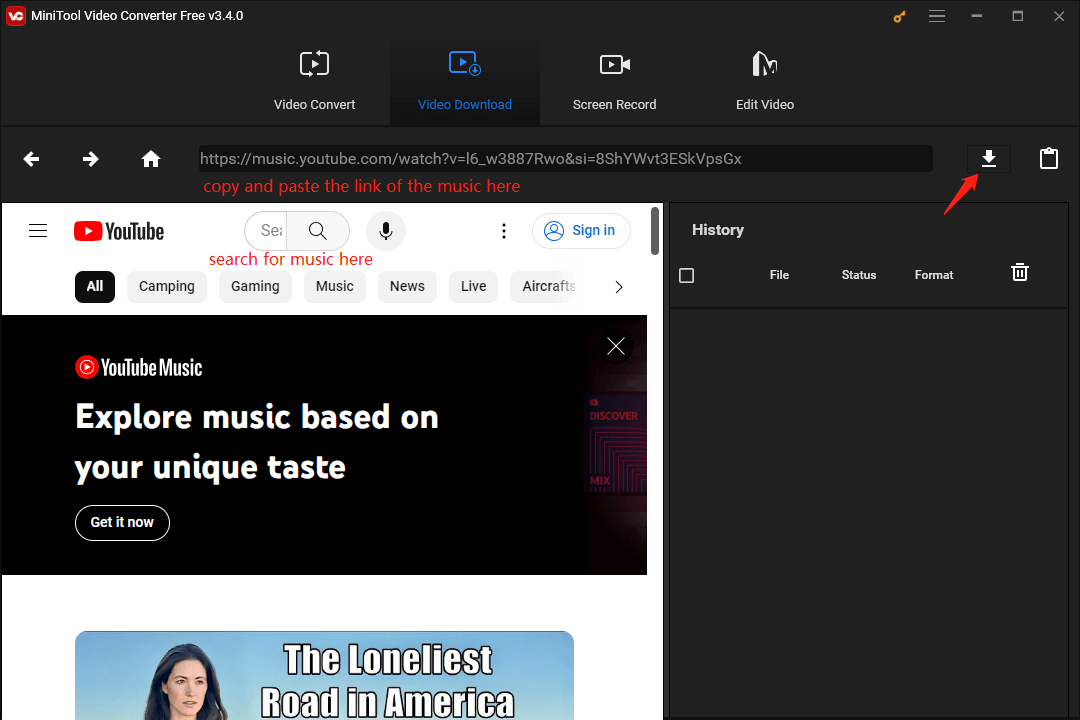In this image, we see a screenshot showcasing the interface of MiniTool Video Converter Free v3.4.0 in the upper left-hand corner. The central section of the interface displays a series of buttons, including 'Video Convert,' 'Video Download' (which is the selected option in this screenshot), 'Screen Record,' and 'Edit Video.' Below this section, on the left side, there are three navigation buttons labeled 'Back,' 'Forwards,' and 'Home.' 

A prominent feature of the interface is a long text box where a YouTube music link has been entered. To the right of this text box, there are two buttons – one for 'Download' and another that appears to be for 'Paste.' Beneath the text box, instructional words have been added, stating, "Copy and Paste the link of the music here," accompanied by a red arrow pointing towards the 'Download' button to highlight it.

On the left side of the interface, there is a section labeled 'YouTube,' with added text indicating, "Search for Music Here." To the right of this, there is another section labeled 'History,' which includes columns for 'File,' 'Status,' and 'Format,' along with a small trash bin icon presumably for deleting entries.